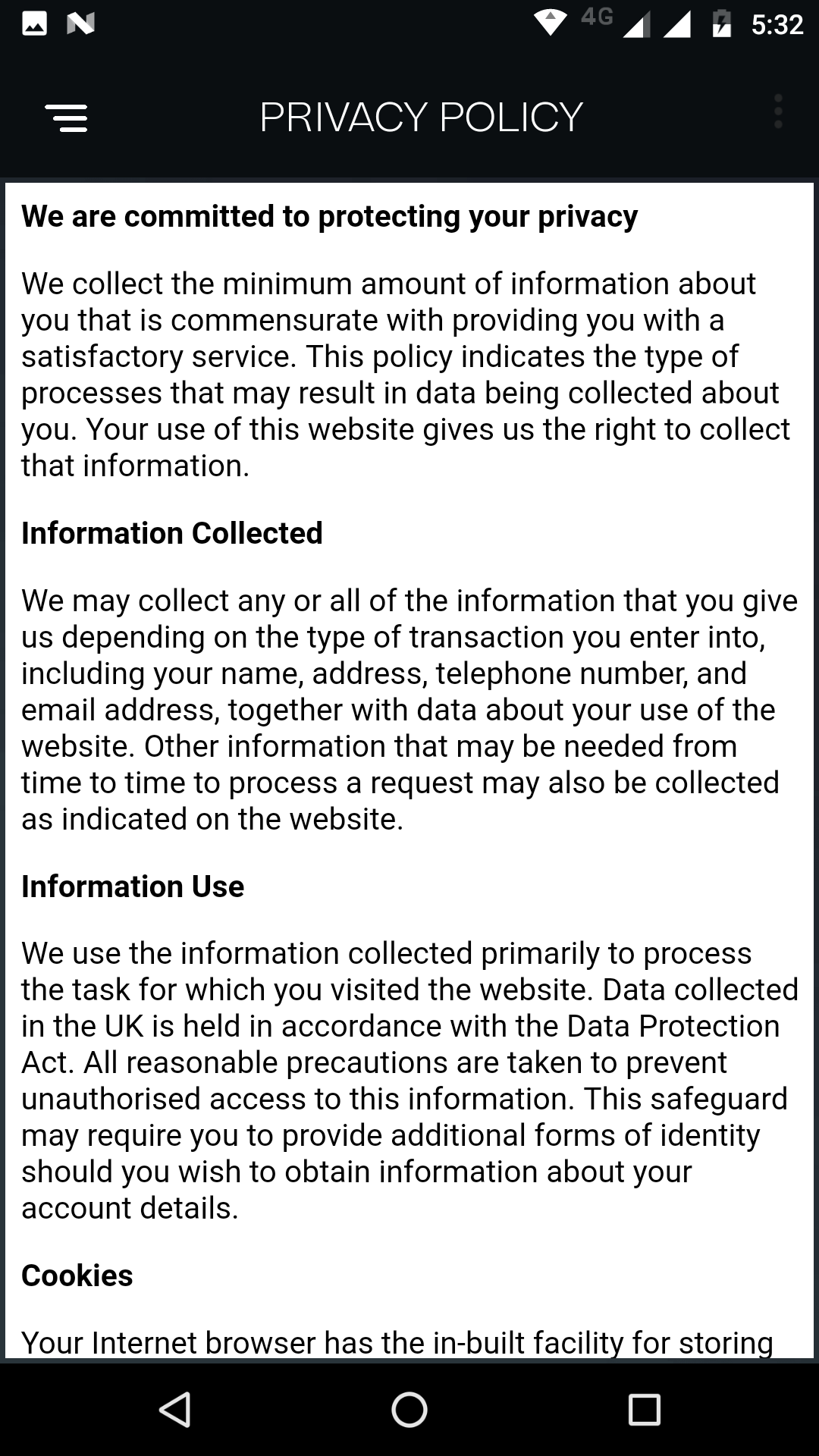This image is a smartphone screenshot showcasing a privacy policy document. At the top of the screen, there is an array of icons from left to right: a photos app icon, a Netflix icon, a Wi-Fi symbol, a 4G indicator, a battery icon at approximately 50% charge, and a timestamp displaying 5:32. On the left side of the screen, there are three horizontal lines, typically indicating a menu. Centered at the top, the title "Privacy Policy" is prominently displayed.

The content of the privacy policy begins with the statement, "We are committed to protecting your privacy." The section titled "Information Collected" follows, repeating the commitment to privacy and stating that the company collects the minimum amount of information necessary to provide satisfactory service. It specifies that the information gathered may include one's name, address, telephone number, email address, and data regarding website usage, depending on the nature of the transaction.

The next section, "Information Use," explains that the collected data is primarily used to process tasks related to the user's visit to the website. Below that is a section on "Cookies," mentioning that the user's internet browser has an inbuilt facility for storing cookies, though the text cuts off abruptly.

The bottom of the screenshot features a black border with a left-facing arrow, a home button, and a stop button.